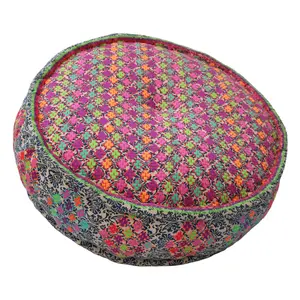This image depicts a realistic-looking, digitally-altered round cushion set against a purely white background, giving it a floating appearance. The cushion appears to feature intricate and colorful designs, possibly inspired by patterns from Asian cultures. The cushion is fairly thick and three-dimensional, suitable for use as a seat or sofa pillow. 

The top part of the cushion showcases vertical stripes with repeating patterns of flowers in hues of purple, pink, blue, green, and orange. These floral images are meticulously detailed, creating a vibrant tapestry effect. Surrounding the cushion is a rim that connects two circular sections, resembling a long, thin rectangular strip encircling the circular top and bottom.

The sides of the cushion are adorned with black and white design patterns interspersed with circular floral clusters of pink, green, purple, and blue. These colorful circular areas are consistently repeated around the edges, creating a harmonious blend of monochrome and vivid floral imagery.